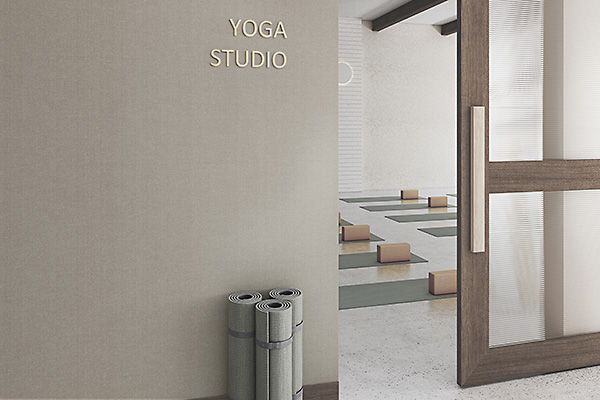The image depicts a professional-looking yoga studio, characterized by a predominantly gray and white palette. Central to the composition is a gray wall bearing the inscription "YOGA STUDIO" in uppercase letters. Below this inscription, three rolled yoga mats, secured with straps, rest against the wall. To the right, a partly opened sliding door with frosted glass inserts and a long metal handle offers a glimpse into the studio's interior. The door slides horizontally rather than having a traditional doorknob mechanism. Inside the spacious, light-filled room, several green yoga mats are spread out on a speckled white and black floor, each equipped with light brown yoga blocks. This well-organized setup suggests readiness for a session of stretching and exercises.